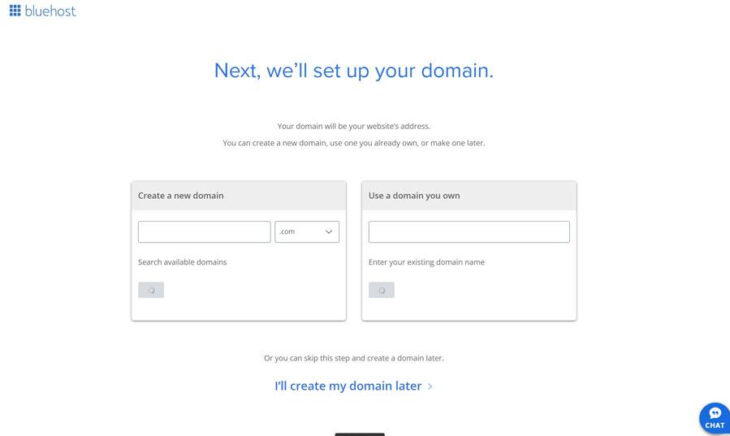The image depicts a webpage from the company Bluehost, with its logo prominently displayed in the upper left-hand corner. The webpage has a clean and professional layout, featuring a prominent blue headline in the center that reads, "Next, we'll set up your domain." Directly below this headline, a small print in black explains, "Your domain will be your website's address. You can create a new domain, use one you already own, or make one later."

In the main section of the webpage, two distinct options are presented in clearly defined boxes:

1. **Create a New Domain**: This section has a gray headline and contains an open input box where users can enter a desired domain name. Adjacent to the input field is a drop-down menu displaying a generic placeholder, "Ibelieve.com," indicating users can choose different domain extensions. Beneath this input field, there is a clickable gray box labeled "Search Available Domains."

2. **Use a Domain You Own**: Positioned to the right, this section features a white input box prompting users to "Enter your existing domain name." Below this input field is another clickable gray box used to search for the existing domain.

Additionally, the webpage offers an option to skip domain setup for the moment, with a blue text link stating, "I'll create my domain later." This user-friendly design ensures that users can proceed with their website setup smoothly, whether they are creating a new domain or using an existing one.